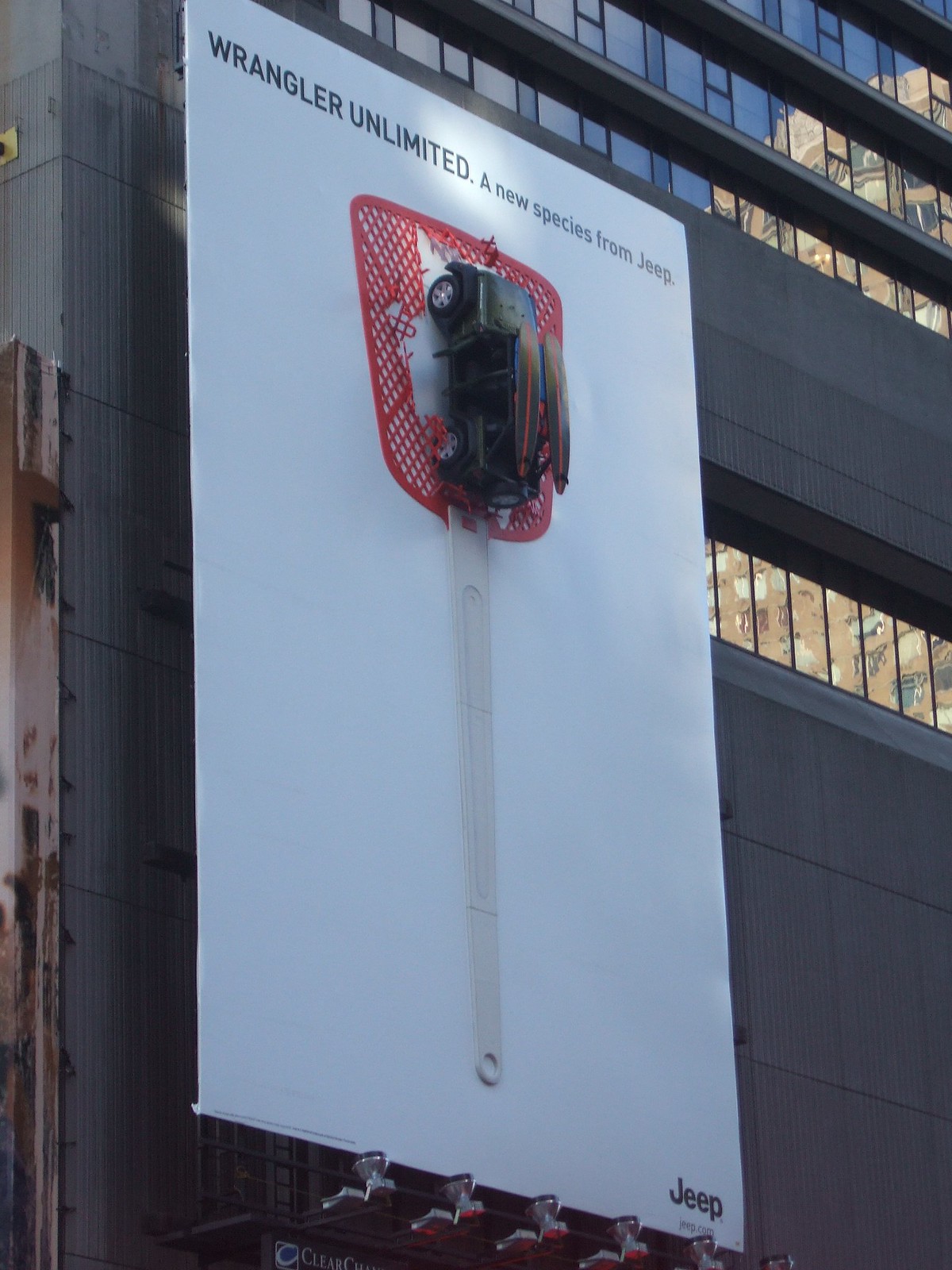The image features a striking advertisement displayed on the side of a modern, gray high-rise office building. The billboard, approximately four stories tall, is the main focus and is designed with a clever 3D effect that integrates seamlessly with the architectural environment. The white billboard prominently displays the slogan "Wrangler Unlimited, a new species from Jeep" at the top in black font. Positioned centrally is a dramatic visual of a unique green Jeep Wrangler, equipped with black surfboards that have orange or red stripes. The Jeep appears indestructible as it breaks through a large, red fly swatter with a white handle. The swatter's top, shattered into pieces, suggests the Jeep's ruggedness and resilience as part of its "new species" branding message. The advertisement is enhanced by a row of spotlights below, likely illuminating the billboard at night, making it a standout feature in an urban setting. Reflections of a tan building can be seen in the high-rise's windows on the left-hand side, adding depth to the scene.